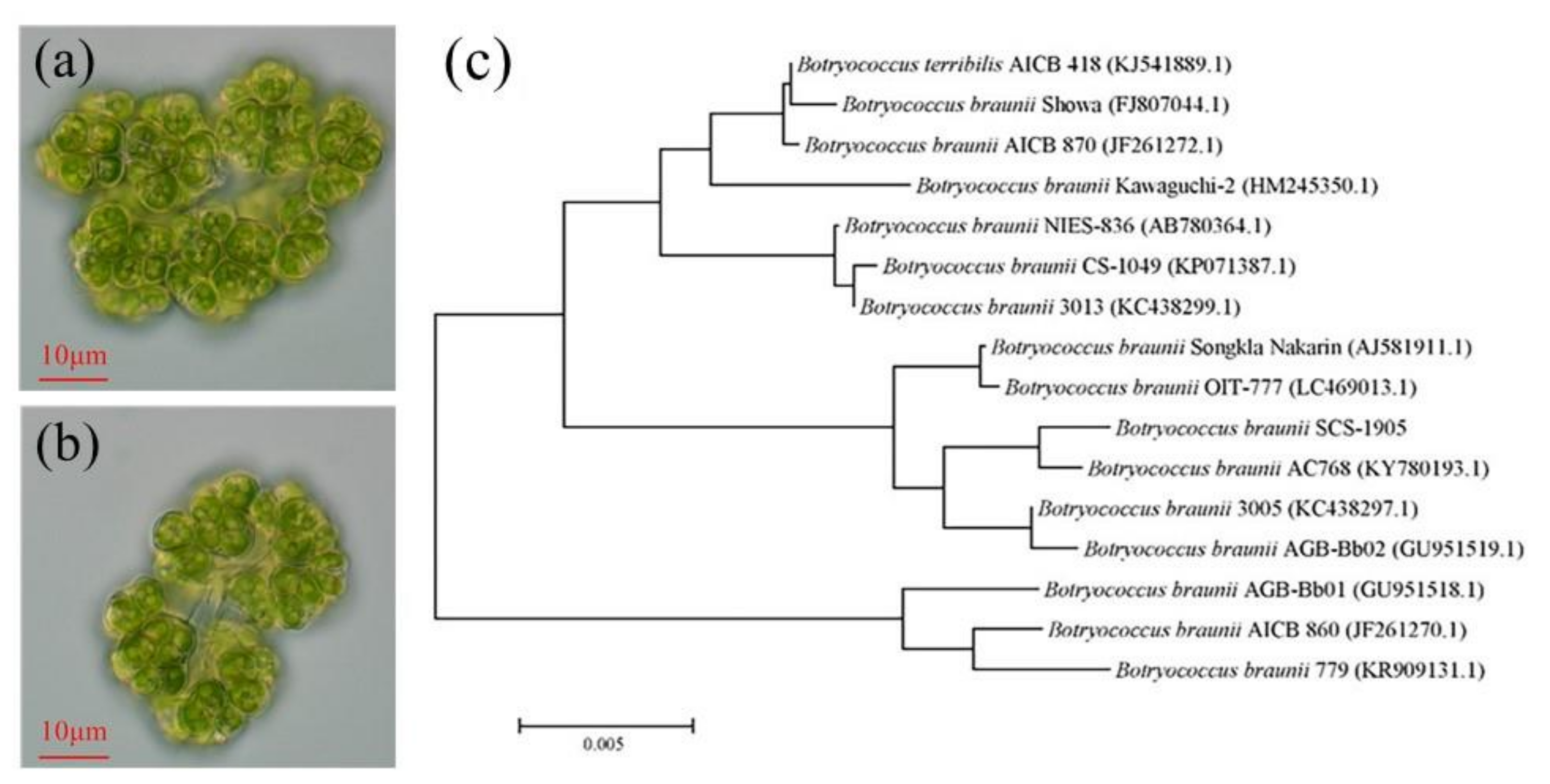The image is a detailed botanical diagram focused on cell morphology, featuring three main sections labeled A, B, and C. In section A, located at the top left, there is an image of a green cell structure with a circular formation, set against a gray background and marked with "10 p.m." In section B, directly below A, a similar green cell structure is depicted but in the process of separating into two parts, also marked "10 p.m." To the right in section C, there is extensive textual information in tiny print, listing various scientific names and identifiers such as "Botryococcus terribilis, AICB418" with additional lines and arrows connecting terms, suggesting a detailed classification or description of the cell structures depicted in the images.